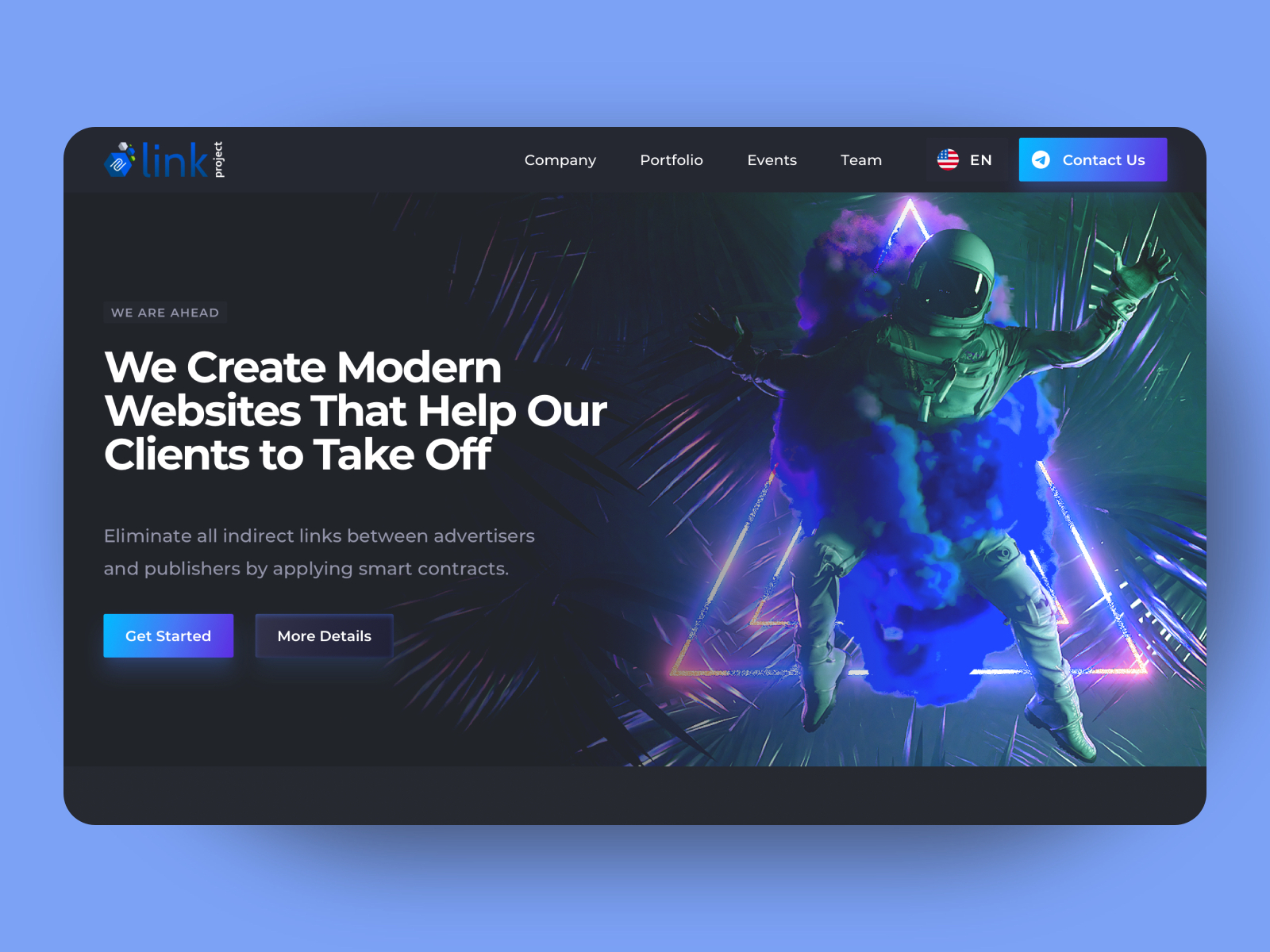This screenshot captures a website's homepage for a company called Link Project. Dominating the top section of the page, the navigation bar features tabs labeled "Company," "Portfolio," "Events," and "Team," alongside an option to change the language and region. A prominent blue "Contact Us" button suggests it is possible to send direct messages.

The background of the page is black, bringing dramatic contrast to a vivid, abstract image nestled in the center. This image features an astronaut surrounded by colorful, smoky hues, primarily blue, with a geometric triangle behind him and palm trees, lending an outer-space yet tropical fusion.

White text overlays the image, reading "We are ahead. We create modern websites that help our clients to take off," which ties into the astronaut's imagery. Further down, it states, "Eliminate all indirect links between advertisers and publishers by applying smart contracts."

Below this text are two interactive buttons: a blue "Get Started" button and a black "More Details" button. Finally, the website is set against a light blue background, adding a subtle yet refined aesthetic to the interface.